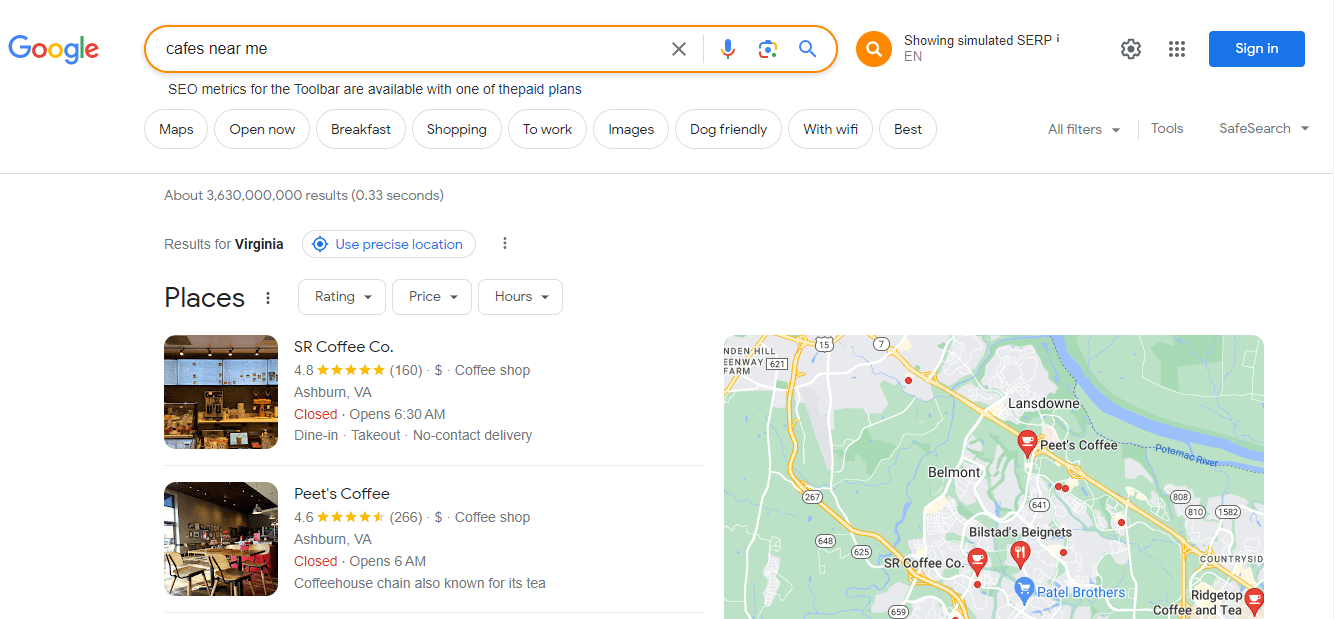The image displays a Google Maps web page specifically designed to help users find nearby cafes. At the top left corner, the "Google" logo is prominently featured. To its right lies the Google search bar, which includes both a microphone icon for voice-activated searches and a text input field where the user has typed "cafes near me." 

Below the search bar, several filter options are available, such as "Open now," "Breakfast," "Shopping," "To work," "Images," "Dog-friendly," "With Wi-Fi," and "Best," enabling users to refine their search results further. 

The search results have yielded two cafes in Virginia. Above the results, there is a prompt in blue text, “Use precise location.” The first listing is for "SR Coffee Co. Company," which boasts a rating of 4.8 stars from 160 reviews and features a single dollar sign indicating its price range. This coffee shop, located in Ashburn, Virginia, is currently closed but set to open at 6 AM. The second option is "Pete's Coffee," rated at 4.6 stars based on 266 reviews, also marked with a single dollar sign. This cafe, known for its tea, is likewise situated in Ashburn, Virginia, and will open at 6 AM.

To the right of the search options and results, a map of the local area is displayed, marking the locations of various coffee shops, including the two listed cafes.